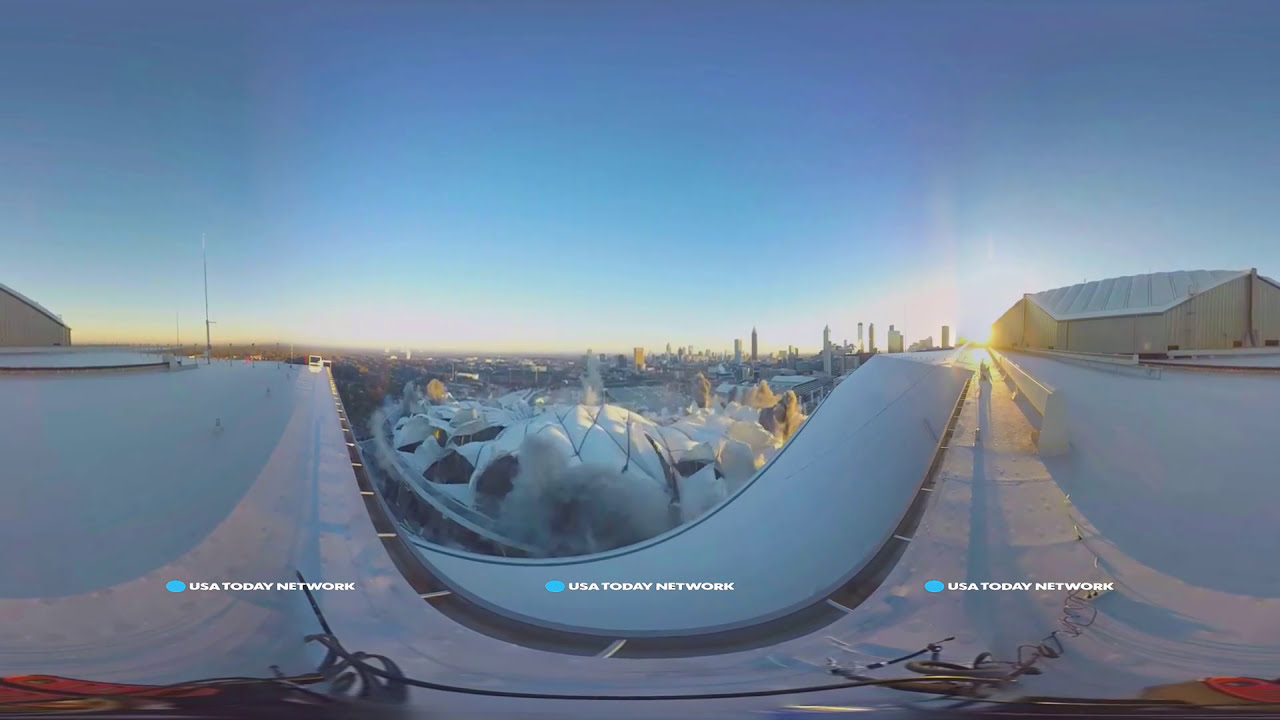In this photograph, we observe a modernistic urban rooftop scene during winter, characterized by a panoramic 360-degree perspective. The foreground highlights a curving rooftop that arches from the left, leading our eyes to a set of domed, tent-like white structures which appear permanent and substantial, emitting smoke from openings. Below this, black lines and rails partially veiled by snow curve and extend, lending a unique texture to the scene.

The background reveals a skyline filled with conventional edifices and skyscrapers, suggesting a city environment. The large tan building to the right, topped with a white metal roof, further accentuates the urban setting. The roof itself bears noticeable line patterns beneath the snow. Adjacent to this building, there is a beige wall with a vertical chimney or exhaust system, contrasting with the snow-covered surroundings.

The entire scene is blanketed in snow, giving it a monochromatic, serene quality with an underlying sense of vivid contrast provided by the blue sky overhead. The sky transitions at the horizon where a sliver of yellow light hints at either dawn or dusk, with the sun brightly shining from behind the structures on the right. Scrawled across the image multiple times is the text "USA Today Network," signaling its source.